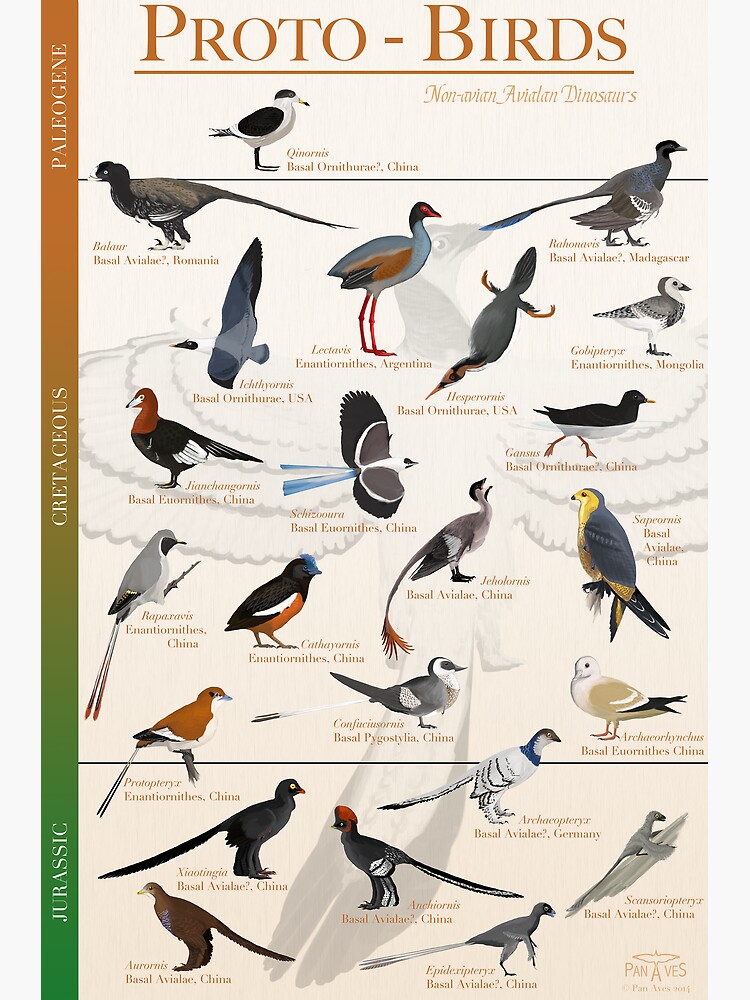This detailed infographic categorized under the title "PROTO-BIRDS" prominently features illustrated drawings of various bird species spanning different geological periods. The subtitle, "NON-AVIAN AVIALIN DINOSAURS," is in cursive beneath the main header. The birds are arranged into three sections based on their historical period: Jurassic, Cretaceous, and Paleogene. Each section, shown on a vertical banner transitioning from green to red to rust color, organizes birds by their time period and provides specific details about each bird, including its name and region of origin. The Jurassic section highlights more dinosaur-like birds, the Cretaceous section features a diverse and colorful array of birds, while the Paleogene section includes fewer, yet distinctly different birds. Many birds originate from regions such as China, Romania, Madagascar, Mongolia, the USA, and Argentina. At the bottom, the label "panvase" indicates the creator of the infographic, which appears to be a detailed, visually rich resource likely sourced from scientific literature or educational materials.